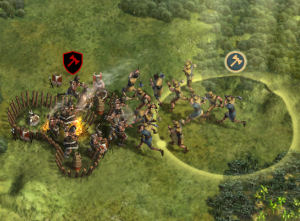This image depicts an intense battle scene from an unspecified video game. In the foreground, a group of warriors or soldiers is engaged in fierce combat within a vast, grassy field dotted with straw and a few scattered trees on the right side. Central to the scene is a cluster of men standing amidst a series of sticks, around which a fire has erupted, casting a dramatic glow. Above these fighters, there is a symbolic shield emblazoned with a red hammer on a black background, possibly representing a faction or emblem within the game.

As the battle unfolds, additional men are seen running towards the central group, contributing to the chaos and urgency of the skirmish. Among these combatants, some are positioned within a distinctive light-green ring that may be a result of sunlight or some other in-game effect, adding an ethereal quality to the scene. Above the melee, a small circle with a blue background and an axe symbol can be seen, perhaps indicating an objective or significant marker in the game. The overall composition suggests a high-stakes confrontation with rich, dynamic visuals and intricate details emblematic of the game's immersive environment.